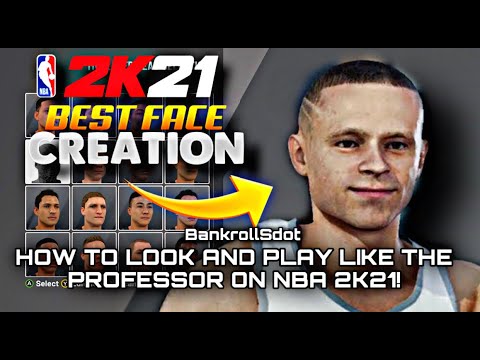Here is a detailed, cleaned-up caption for the image described:

---

Screenshot of a digital interface on either a PC or tablet displaying an app for creating AI-generated human faces. The interface appears sophisticated and is illuminated on a dark background with a black border on the top and bottom; the central section is gray. Dominating the right side of the screen is a photo or graphic of a young, light-skinned, biracial man with closely shaved hair, smiling warmly. He is dressed in a white singlet with gray trim.

To the left of this image, prominent large text features the NBA logo followed by "2K" in red, "21" in white, and underneath, in yellow text, "Best Face." Further down, in white, it says "Creation." The combination of these elements reads: "NBA 2K21 Best Face Creation." Below this, a large yellow arrow points towards the man's image, emphasizing the heading in bold text: "How to Look and Play like the Professor on NBA 2K21." 

Inset into the background underneath the main text is a faint template displaying various faces, suggesting options for customization within the app.

---

This cleaned-up caption conveys all the important details while providing a clear and cohesive description of the image.